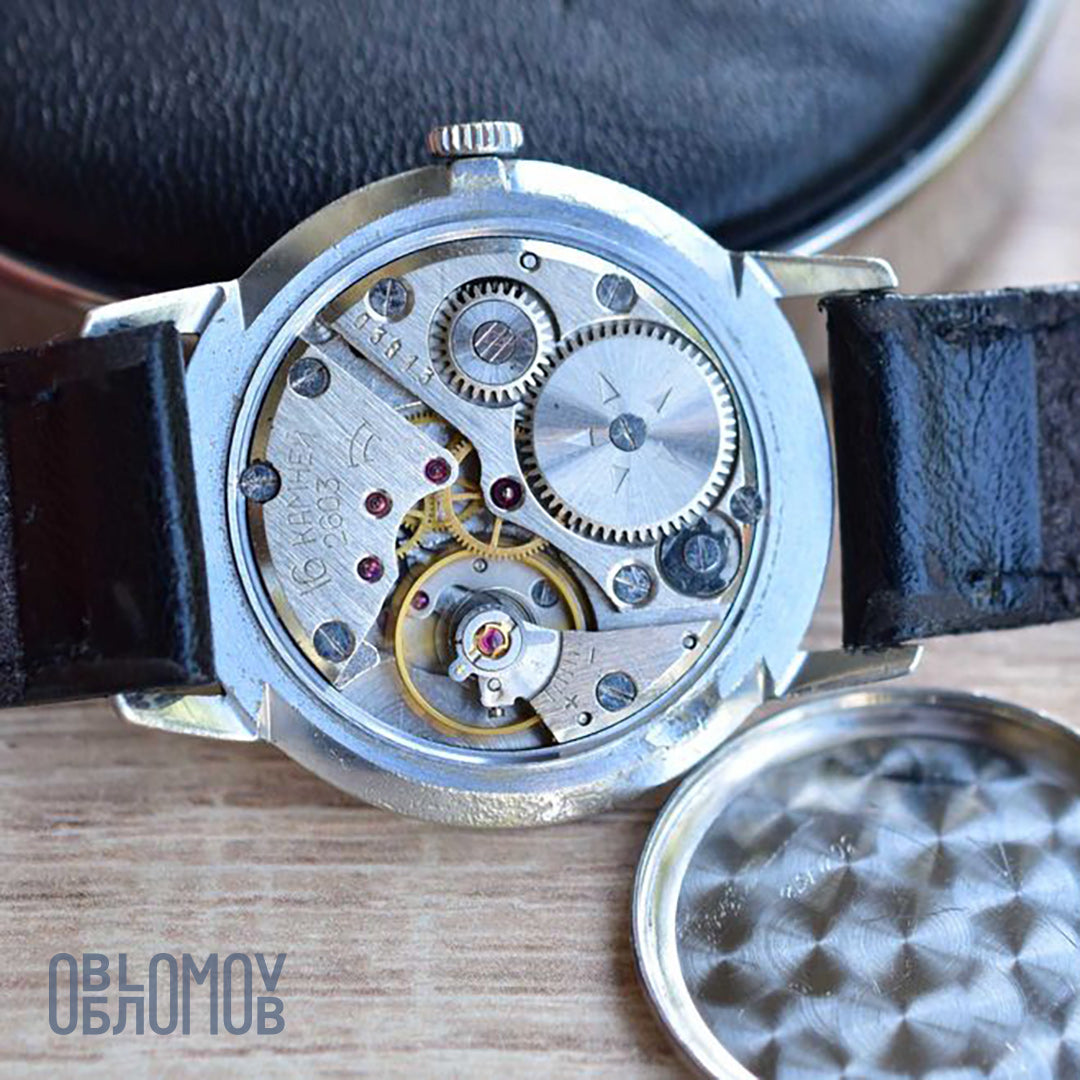This photograph vividly showcases the intricate back of a fine wind-up watch, emphasizing its elegant engineering and detailed craftsmanship. The watch features a black leather band and rests on a wooden tabletop, accentuating its sleek, silver-colored casing, potentially stainless steel. The image highlights the innards of the watch, with three prominent dials and several smaller ones beneath them, showcasing the mechanical finesse and functional beauty of the timepiece. The back cover, laying beside the watch, reveals an etched pattern, adding to the intricate detailing. Notably, screws are visible, securing the various components together. In the bottom left corner of the photo, there are some non-English letters, further hinting at the watch's distinguished craftsmanship and possibly indicating a brand name. The zoomed-in perspective focuses on the watch's plate, offering an engaging view of the cogs and moving parts that are rarely visible in most timepieces.